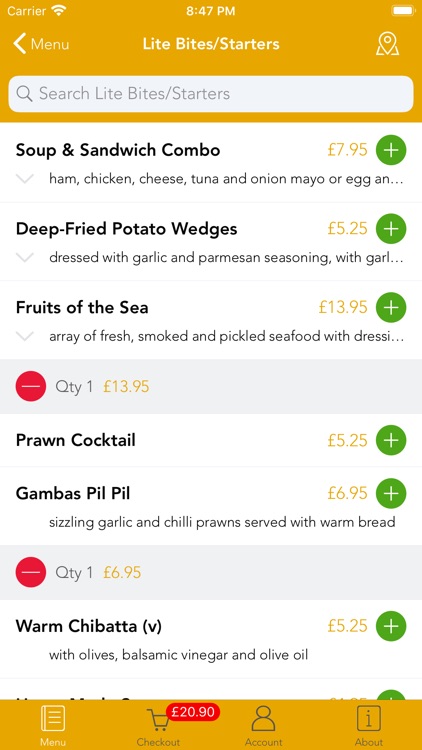This is a screenshot from a menu app on a smartphone. At the top, the header features a dark yellow background. Centered within the header is the text "Light Bites Starters" in bold white font. On the left side of the header, there is the word "Menu" in small white font, accompanied by a leftward-pointing arrow. On the right side, there is a location icon. Just below the header, there is a search bar that reads "Search Light Bites Starters."

The body of the app menu has a white background and lists menu items vertically. The first item at the top left is "Soup and Sandwich Combo" displayed in bold black font. To the right of this item, the price is shown in red, along with a green circle containing a plus sign to add the item to your bag. Below that, under the section labeled "Fruits of the Sea," the quantity is marked as one. Further down the page, under "Gambas Pil Pil," the quantity is also listed as one.

At the bottom of the screenshot, there is a dark yellow bar. On the left side of this bar, the "Menu" option is highlighted in white. To the right of that, there's the "Checkout" option, which displays a total of $20.90 in a red circle at the top right of the icon. Also visible are the "Account" and "About" options.